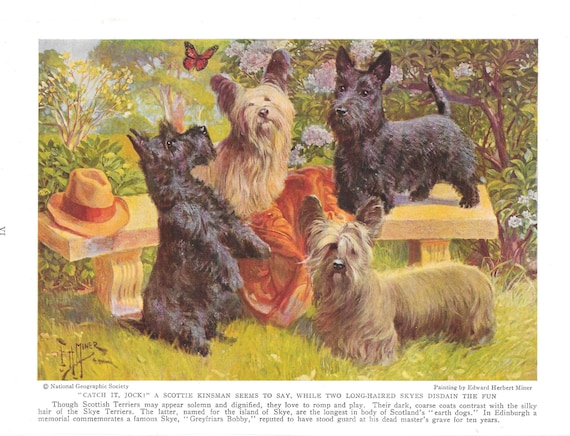This illustration by Edward Herbert Minor, titled "Catch it, Jock," is a vibrant depiction of four dogs, rendered in a colorful and detailed style. At the bottom, the image is attributed to the National Geographic Society. The scene captures the playful interaction of two Scottish Terriers and two long-haired Skye Terriers, who appear to be observing an orange monarch butterfly fluttering nearby. The Scottish Terriers, known for their solemn and dignified demeanor, are shown enjoying a moment of playful curiosity, contrasting with the Skye Terriers' distinguished silky coats and longer bodies, characteristic of the breed named after the Isle of Skye. The illustration references a beloved story from Edinburgh about Greyfriars Bobby, a Skye Terrier famously loyal to his deceased master, commemorating his ten-year vigil at his master's grave with a minute memorial. The dogs stand on lush green grass with trees providing a serene backdrop, adding to the picturesque and whimsical nature of the illustration.